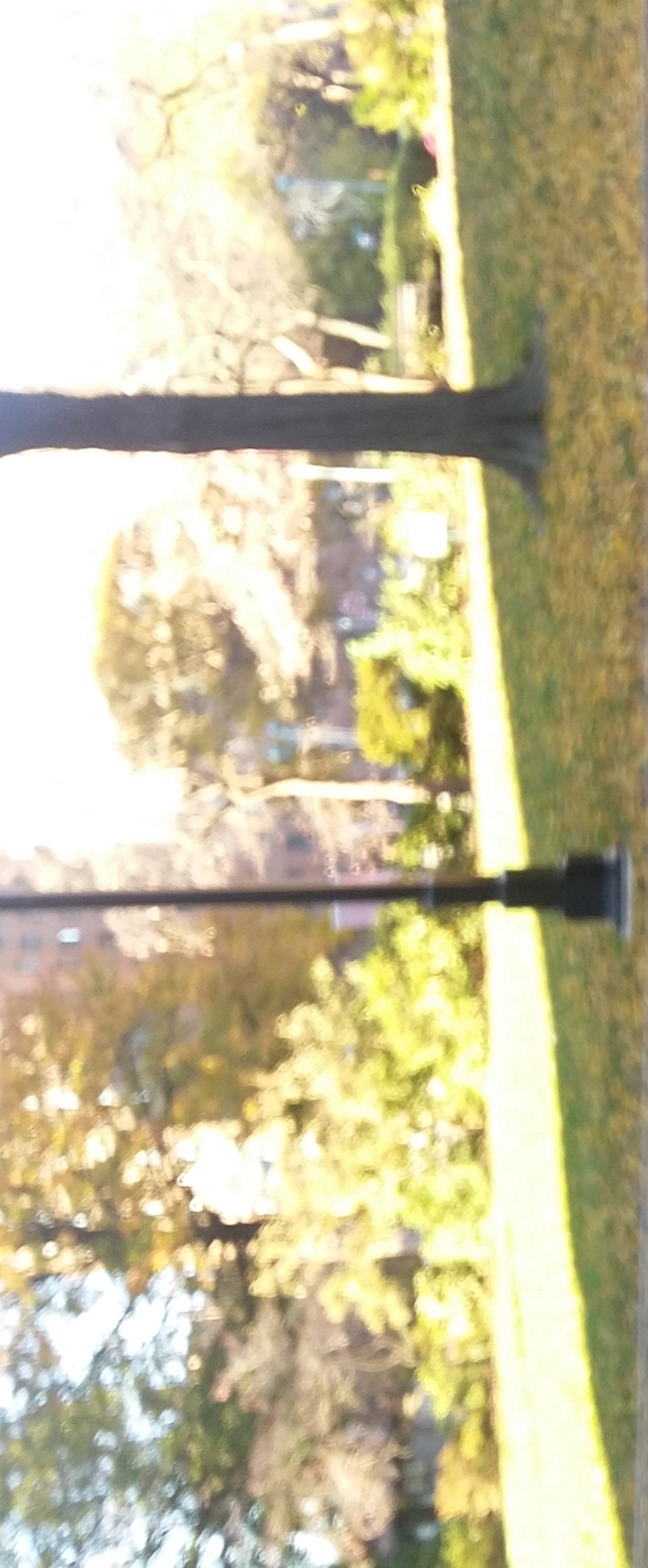In this low-resolution, rectangular photograph taken in daylight, we observe an outdoor scene bathed in bright sunlight. A winding path stretches from the lower left to the right of the image, gleaming under the sun's rays. Beyond the path, a line of bushes and trees forms a natural barrier. Despite the image's graininess obscuring finer details, two objects are discernible on the grassy area in the lower right corner. To the left of this section stands the base of what appears to be a black streetlight, and to its right, the trunk of a tree emerges, though only the trunk is visible in the frame.